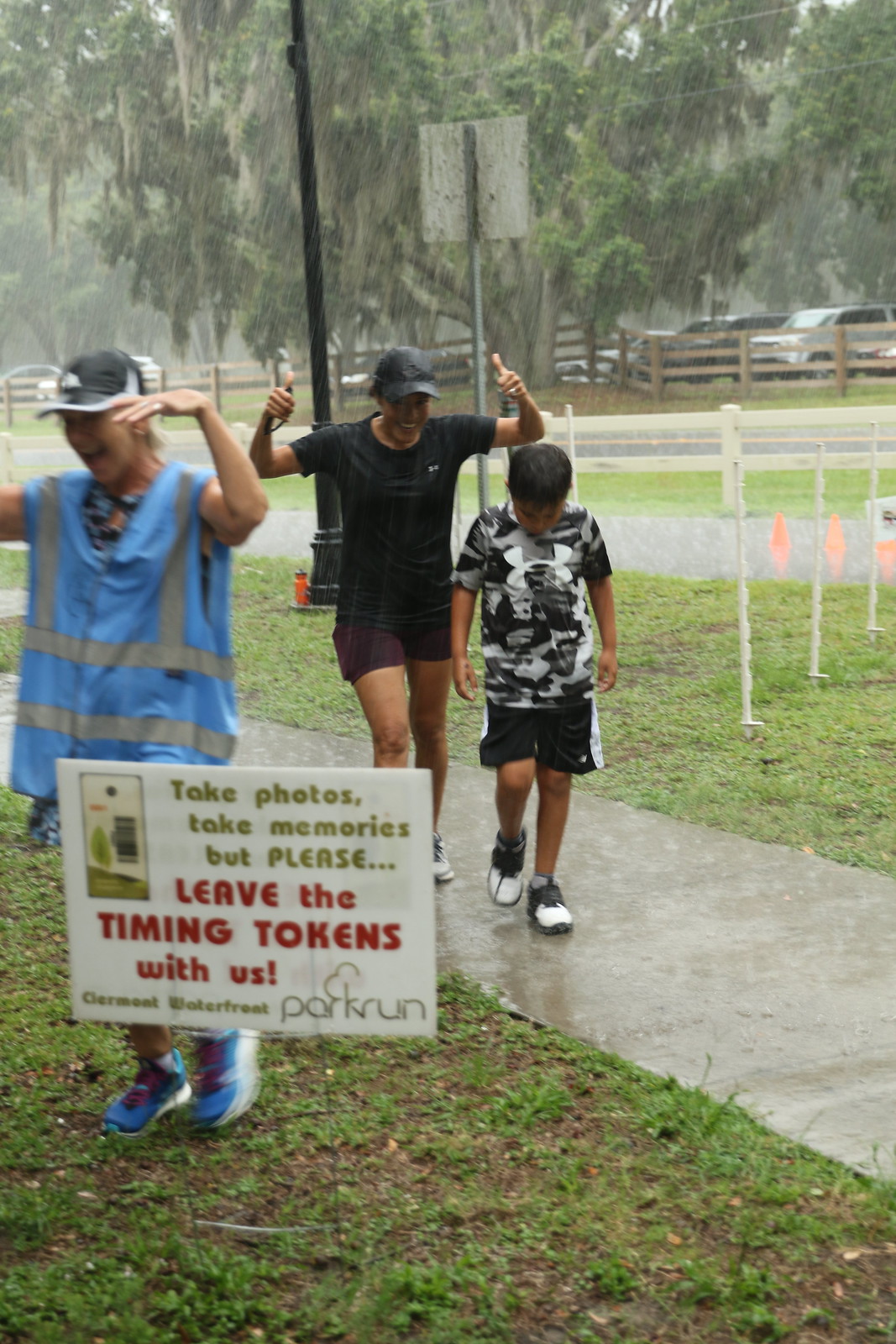In this outdoor photograph taken during heavy rain, three individuals are captured against the backdrop of a parking area with several vehicles and a large tree. In the foreground, a sign on the left reads "Take photos, take memories, but please leave the timing tokens with us" in green and red lettering, accompanied by the "Garment Waterfront Park Run" logo.

The trio consists of: an adult woman on the far left, standing on the grass and wearing a black cap, a red vest over her blouse, and white, blue, and pink shoes. She has her hands outstretched towards the sides. To her right, a medium-complexioned woman in cranberry shorts and a black shirt with a black cap, giving a thumbs-up gesture with both hands. Next to her is a young boy, approximately 8 to 12 years old, dressed in black shorts and a gray and white camo-patterned t-shirt with an Under Armour logo, looking down at the ground. The main colors in the scene are green, blue, white, and black. The setting features a zig-zagging wooden fence and multiple posts, with water visibly accumulated on the ground, and a distant water reservoir near the road.